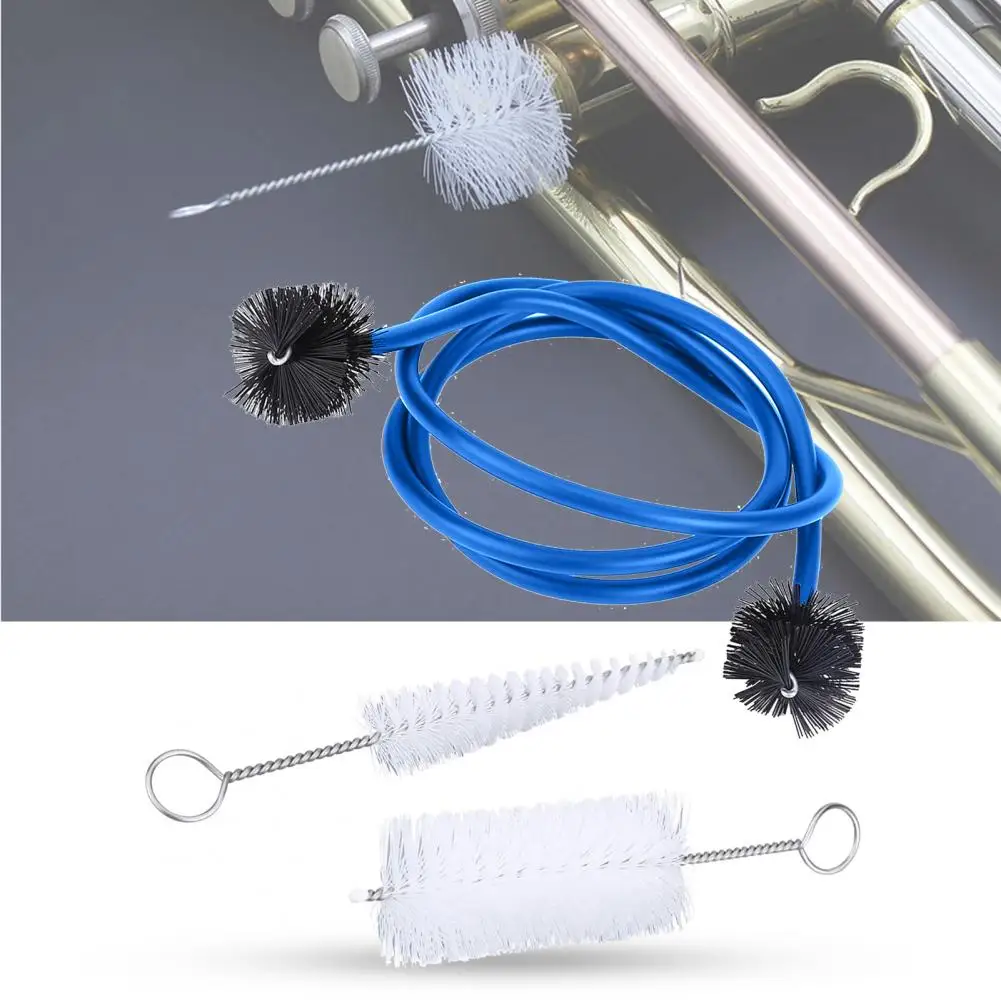This detailed image showcases an array of specialized instruments designed for cleaning brass musical instruments. Prominently featured at the top is a brass instrument lying on its side, with a white coiled brush inserted into one of its embouchures. Below it is a blue, flexible tube-like instrument, which has black bristles on either end and is coiled upon itself. Further down in the image are two silver-handled brushes with white bristles, closely resembling the brush inside the brass instrument. Despite their resemblance to pipe cleaners or even toilet brushes, these tools are specifically crafted for instrument maintenance, effectively reaching and cleaning the intricate internal parts of brass instruments. In the background, metallic pipes can be seen extending outwards, adding to the industrial feel of the scene and emphasizing the detailed nature of the cleaning tools displayed.